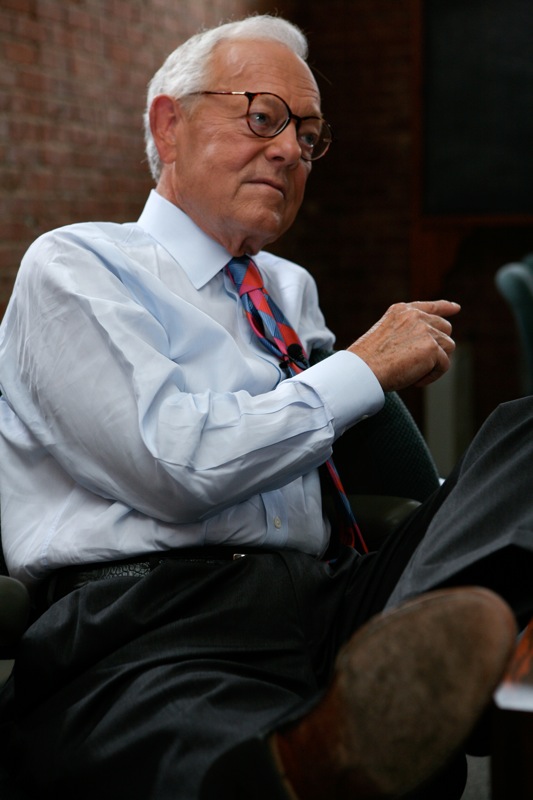The image depicts an older, distinguished gentleman, approximately 70-75 years old, sitting composedly with his left leg crossed over his right knee. He is dressed in a light blue button-down shirt paired with a vibrant red and blue tie, dark trousers, a black belt, and worn dress shoes. His neatly combed white hair and black circular eyeglasses add to his professional appearance. The man appears to be engaged in conversation, glancing to his left, possibly addressing an audience. Behind him, the setting includes a somewhat blurred brick wall showing signs of wear with whitish areas, and a chair back is visible to his left against this backdrop. The overall atmosphere suggests a poised and professional demeanor.